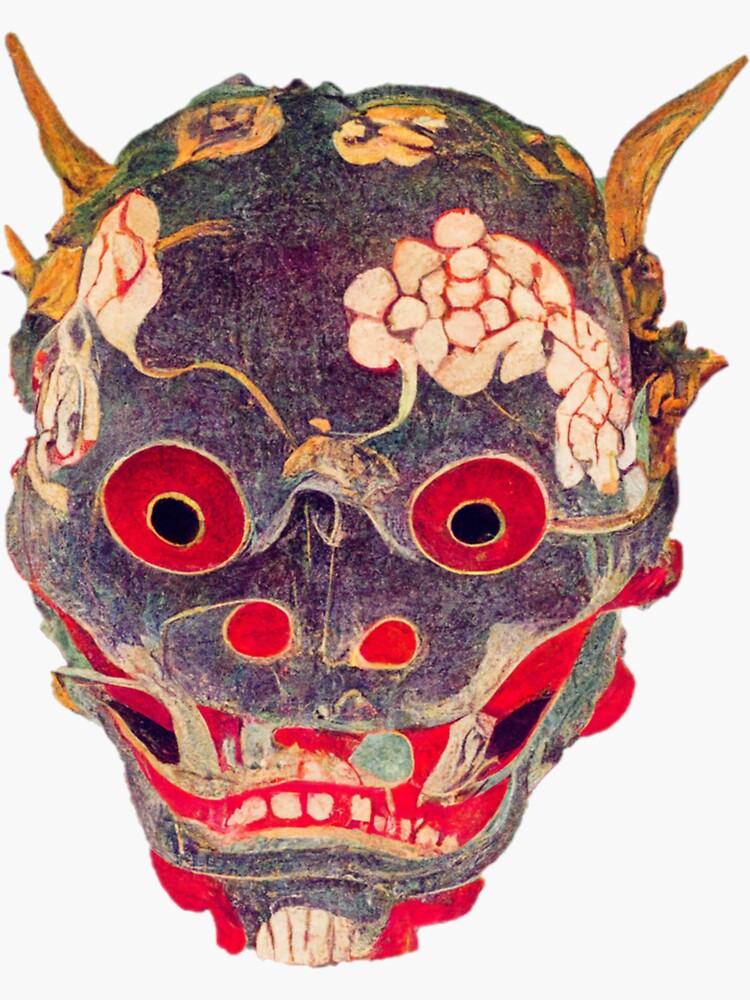This image features an ornate and traditional Asian mask, likely Japanese, potentially used in ceremonial contexts or Kabuki theater. The mask, depicted with a frightening appearance, closely resembles a devil's head or dragon, showcasing sharp teeth that jut out menacingly. It has a striking bluish-purple complexion adorned with light-colored floral motifs. Prominent red eyes with black pupils add to its intimidating look, while the mouth, highlighted in red with hints of gold teeth, appears somewhat abstract and deformed. Completing the mask's menacing visage are orange, albeit rather small, horns perched atop its head. The overall design is highly detailed and visually complex, intricate with various elements that emphasize its traditional and possibly ritualistic purpose.